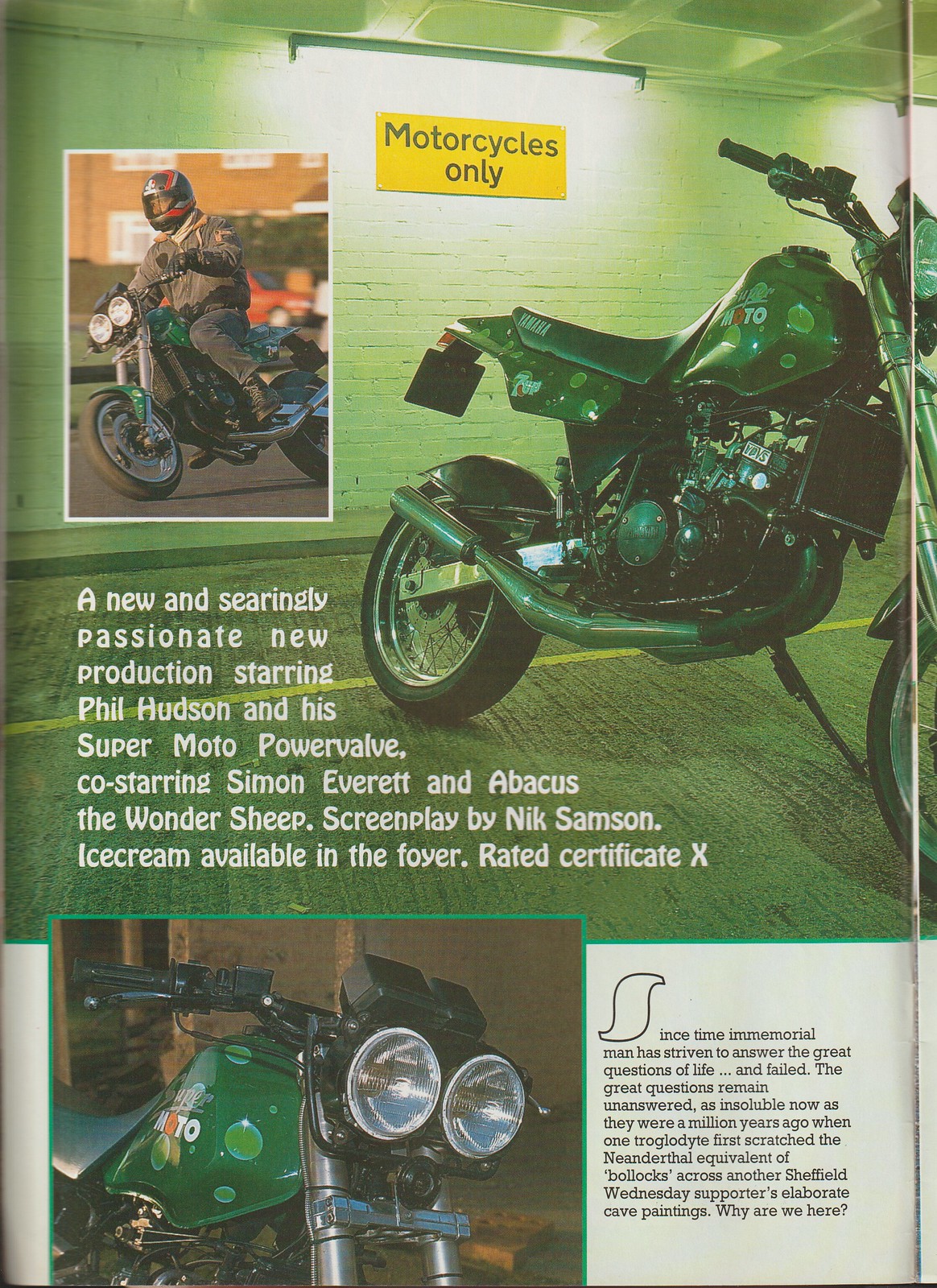The image features a detailed advertisement for a new motorcycle, prominently displayed in a scene dominated by green hues. The main visual focuses on a green motorcycle, set against a brick wall adorned with a yellow sign that reads "Motorcycles Only." The motorcycle's front tire is out of frame, but the visible sections, from the handlebars to the rear, are meticulously showcased. Additionally, there is an inset photo on the left side depicting a man riding this very motorcycle, dressed in riding gear.

The caption below this inset highlights a new and searingly passionate production starring Phil Hudson and his Super Moto Power Valve, co-starring Simon Everett and Abacus the Wonder Sheep. The screenplay is written by Nick Sampson. The advertisement, intriguingly rated Certificate X, mentions that ice cream is available in the foyer.

At the bottom of the advertisement, a close-up image captures the front headlights and a portion of the motorcycle's gas tank. An evocative passage at the bottom left of the advertisement contemplates the timeless existential question of why we are here, poetically linking humanity's enduring search for meaning to ancient cave paintings.